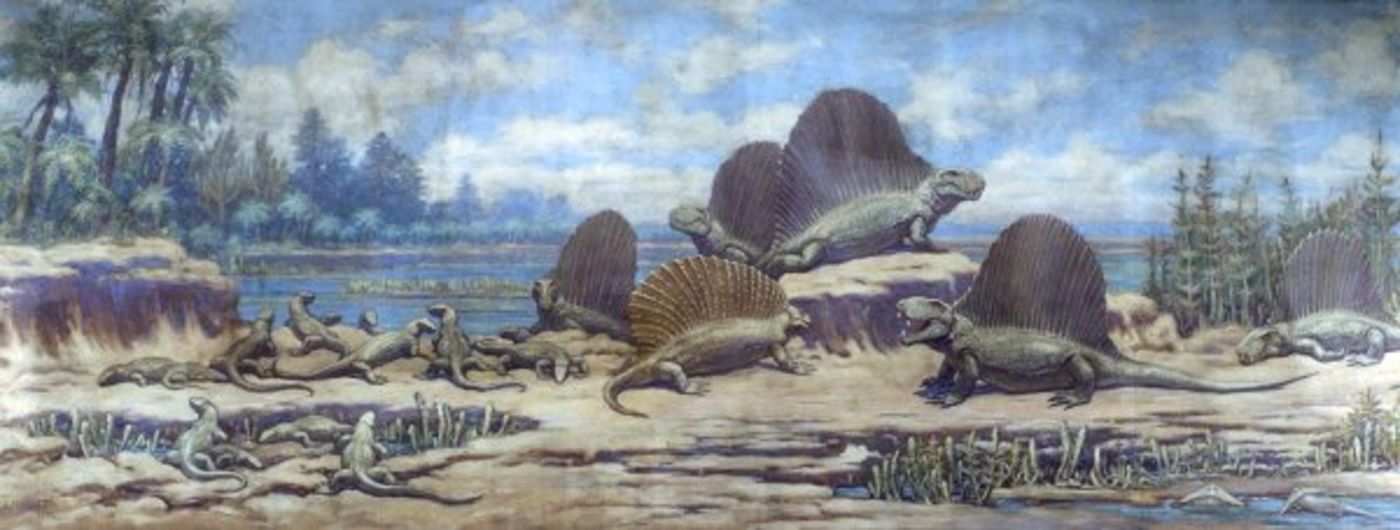The image is a detailed painting depicting a vibrant prehistoric scene, showcasing both the diversity and the grandeur of dinosaur life during the Cretaceous or Jurassic periods. In the foreground, a group of approximately 10 to 15 dinosaurs is gathered, varying in size from imposing adults to tiny babies. One prominent dinosaur, possibly the leader, is perched on a rock, surrounded by others basking in the sunlight on a rocky flatland. These dinosaurs are characterized by large, protruding fans along their spines and some have their mouths open with teeth visible, as if roaring. The background features a picturesque landscape with a blue sky filled with white clouds, a water body, and a lush green forest composed of palm trees and taller evergreen trees, all bathed in warm daylight.